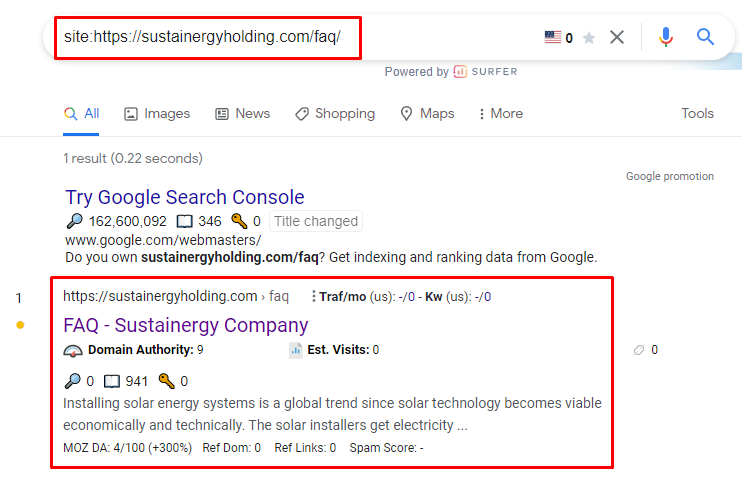This is a screenshot of a web browser displaying search results from the Sustain Energy Holding website's FAQ page. At the top of the browser window, a red search bar features the URL "https://sustainenergyholding.com/faq/" on the left and an American flag along with several computer icons on the right. Below this, a small line of text reads "Powered by Surfer."

The main content area starts with navigation options labeled "All," "Images," "News," "Shopping," "Maps," "More," and "Tools." Underneath, a search result information line shows "1 result (0.22 seconds)." The first result is highlighted in blue text with a link titled "Try Google Search Console," followed by the number "162,600,092."

Further details provide the URL "www.google.com/webmasters" with a prompt reading, "Do you own sustainenergyholding.com/faq? Get indexing and ranking text from Google." 

Below this, a box outlined in red displays the website name "sustainenergyholding.com" followed by "FAQ / Sustain Energy Company" in purple text. The content under this heading discusses domain authority and estimated visits. It also includes a brief excerpt about installing solar energy systems, mentioning the increasing global trend and the economic and technical viability of solar technology, but cutting off mid-sentence: "Installing solar energy systems is a global trend and as solar technology becomes economically and technically viable, the solar installers get electricity..."